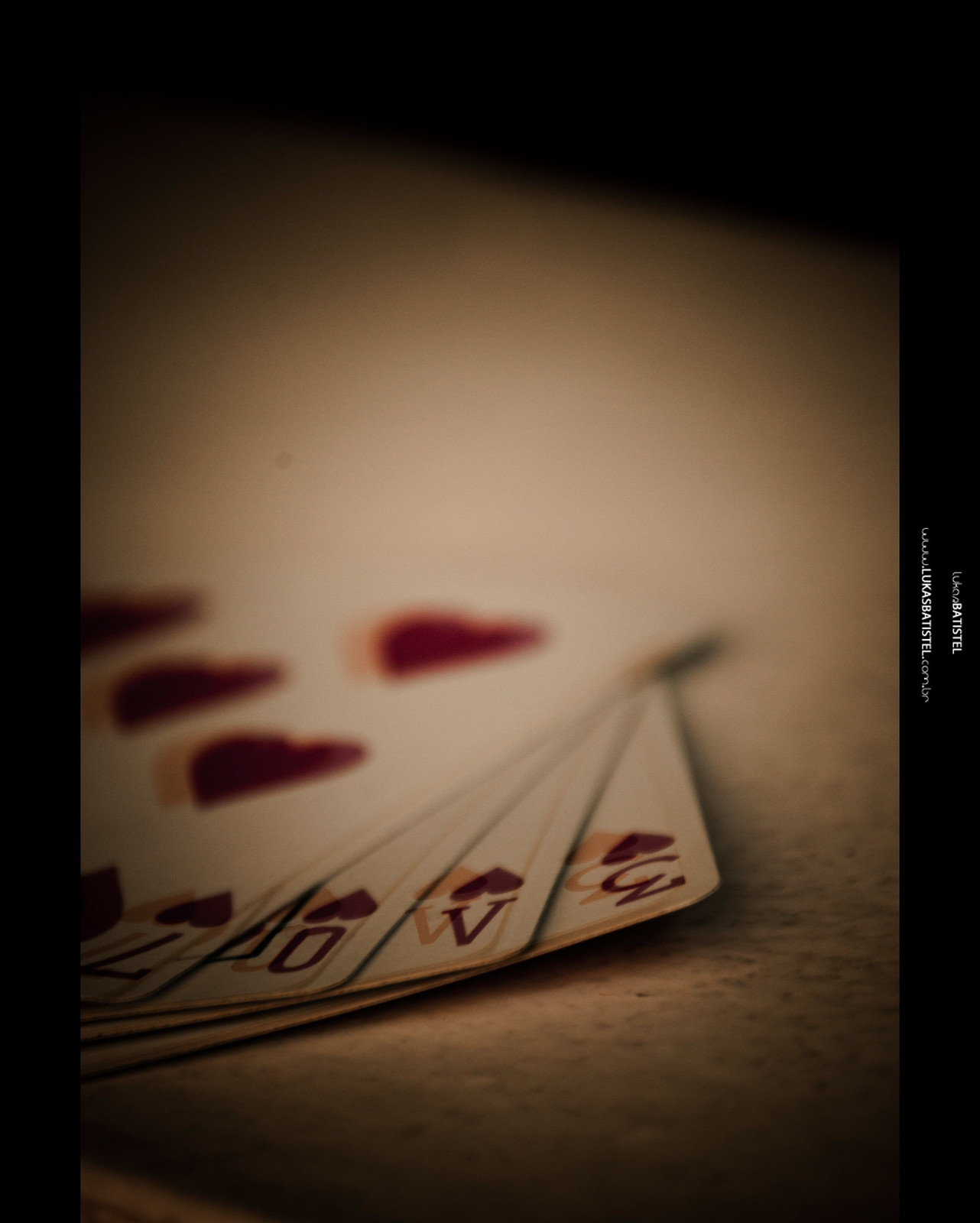This photograph captures a hand of playing cards, all belonging to the suit of hearts, artfully fanned out on a speckled, light-colored surface. Each card features a striking double image: the heart symbol and the number of the card appear in both dark, bold text and a lighter, off-center shadow, creating a unique visual effect. Notably, the "3 of Hearts" card stands out with its dual designations. The background of the image is intentionally blurred, directing focus towards the detailed design of the cards. The picture is framed by a black border that accentuates the central composition.